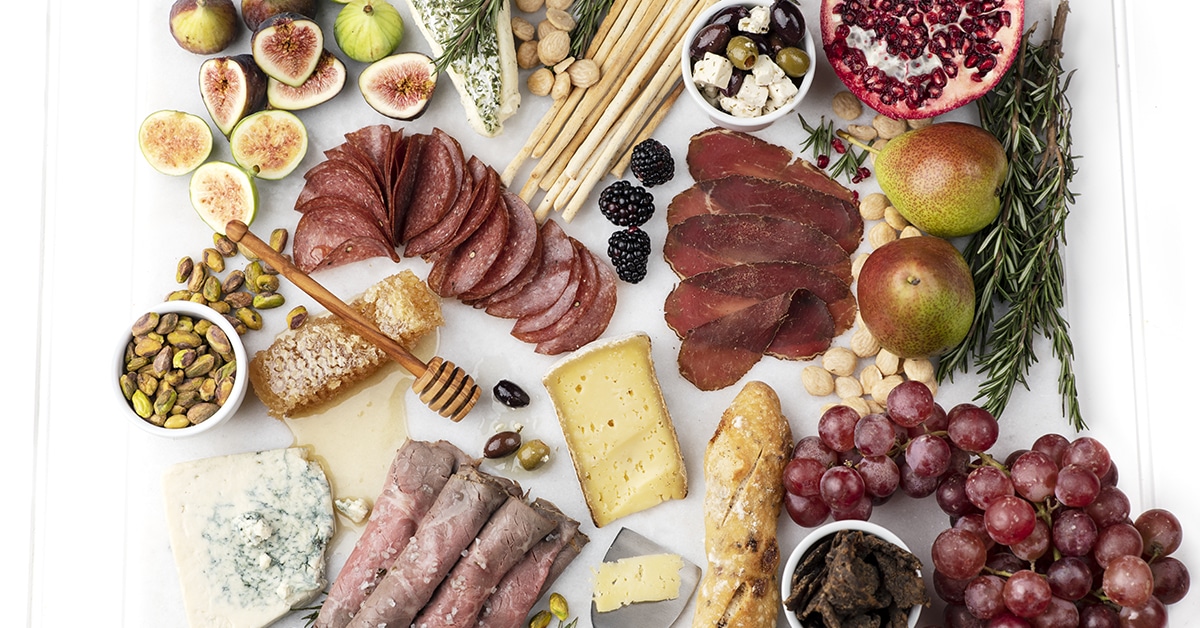The image is a color photograph in landscape orientation, featuring an elaborate cheese party spread displayed on a white tabletop. The arrangement of items, though lacking overt organization, forms a visually appealing assortment of various foods. Positioned centrally are several kinds of cheeses including a prominent piece of blue cheese with a slice cut out using a small spatula. Adjacent to this is a large loaf of bread and a dish of pistachios, with a honey dipper resting on a honeycomb nearby. 

To the right, a selection of meats such as thinly sliced prosciutto, salami, and rolled-up ham pieces are paired with a few blackberries. A cluster of red grapes sits in the bottom right corner alongside a small white dish. Interspersed among these items are assorted nuts including macadamia and chestnuts, and fruits such as pomegranate halves, figs, kiwis, blackberries, and pears. 

Green and red olives are garnished with cubes of feta cheese in a round dish located at the top right, complemented by sprigs of rosemary and bamboo breadsticks. Additional details include kumquat slices and various other cheeses like Swiss cheese. The photograph captures a realistic and detailed representation of a food spread typical for a cheese party, characterized by its vivid colors and diverse selection of items.